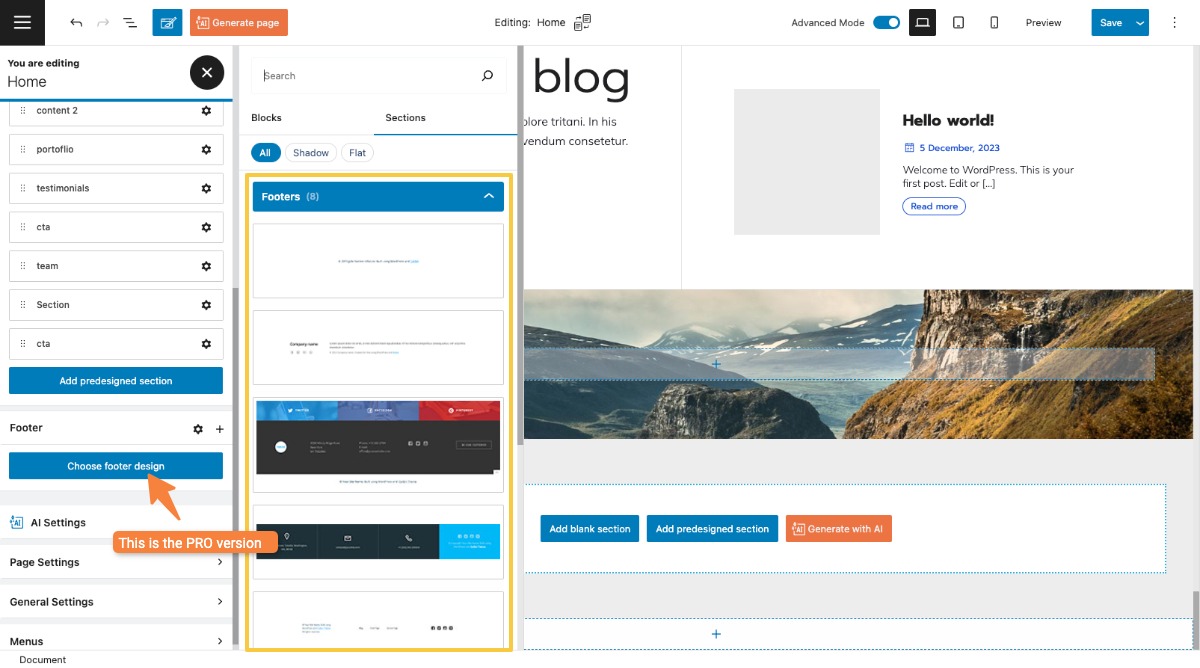This screenshot captures a web page guide for using a web application, specifically a website builder that utilizes block sections for constructing web pages. The image is overlaid with highlighted sections and instructional information, guiding users on where to click and how to operate the application. At the top of the interface, icons for previewing the site and saving progress are visible. A mode toggle allows the user to switch between desktop and mobile phone views. The top right-hand section indicates that the user is currently in edit mode, working on the home page of the site.

On the left-hand side, a design navigation menu offers various settings adjustments. The second block section on this side displays a pop-out menu that lets users delve deeper into the functional sections. The right-hand side’s third block shows a preview of the website being built—currently featuring a blog with an image of a picturesque mountainous scene.